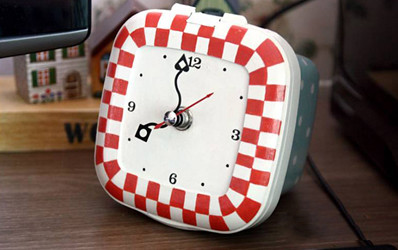This photograph captures a detailed scene set on a dark brown wooden desk. At the center of this composition is an electric clock, distinguished by an evident wire trailing from its base. The clock features a rounded square shape with an eye-catching border of red and white checkered pattern. Its dial is stark white with bold, black numbers, and the time displayed is precisely 8 o'clock with the second hand resting at 7 seconds past the minute. 

In the background, the edge of a computer monitor is partially visible in the left-hand corner, hinting at a busy workspace. Adjacent to the clock, a small wooden sign is placed on the desk, displaying the letters "WA." Atop this sign sits a collection of miniature house models, with one particularly standing out in white, accented with green shutters and red window panes, adding a touch of charm and color to the scene. To the right side of the clock, a television screen occupies the space, completing the multi-functional purpose of the desk setting.